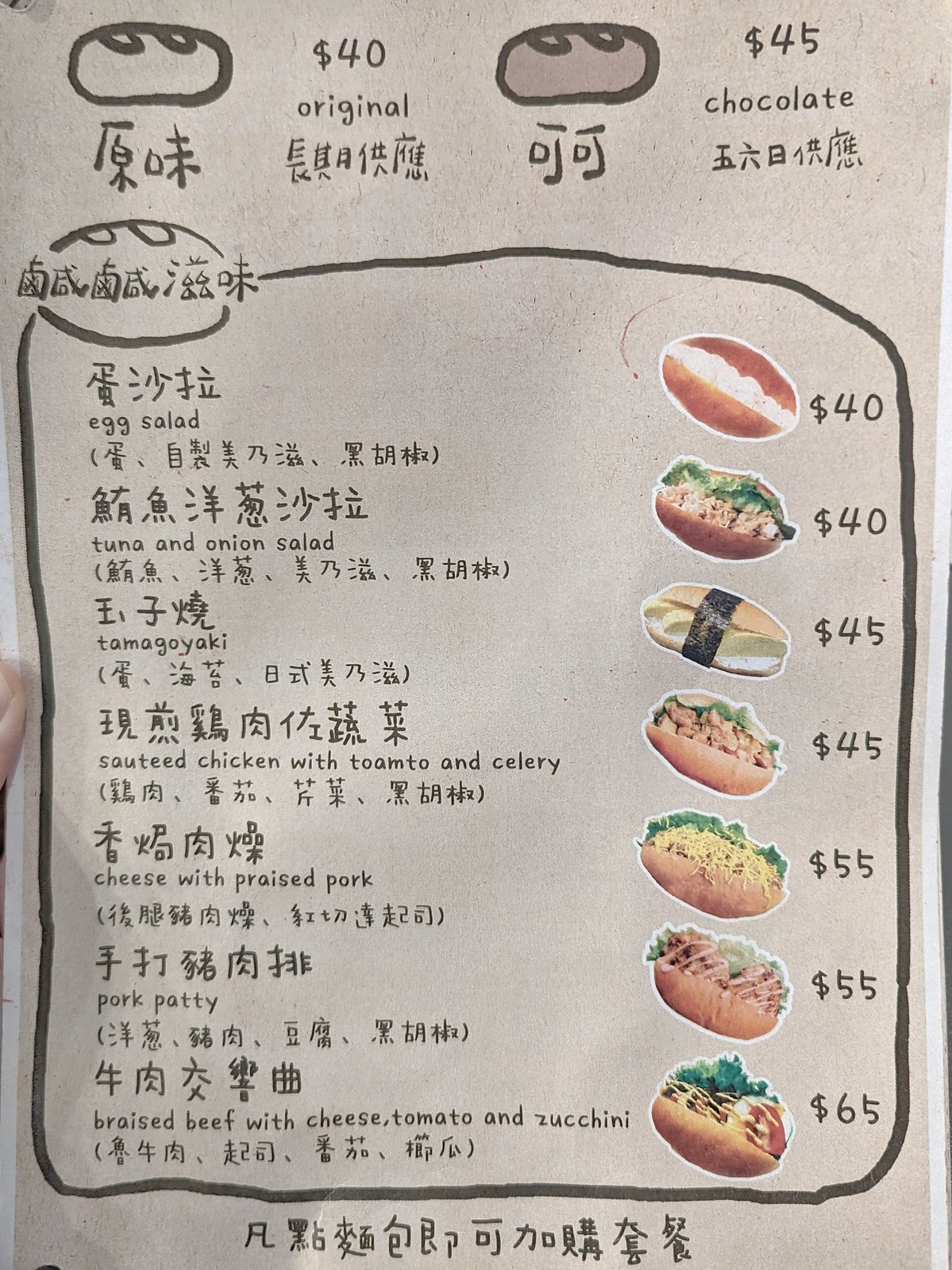The image depicts a bilingual menu presented in both Chinese and English, with a sleek gray background. At the top, there are images of two types of bread: one labeled as "Original" priced at $40, and another as "Chocolate" priced at $45, with corresponding Chinese characters beneath each description. 

The main section of the menu lists various dishes along with their prices and images. The items are detailed as follows:

- Egg Salad priced at $40.
- Tuna and Onion Salad priced at $40.
- Tamagoyaki priced at $45.
- Sautéed Chicken with Tomato and Celery priced at $45.
- Braised Pork priced at $55.
- Pork Patty priced at $55.
- Braised Beef with Cheese, Tomato, and Zucchini priced at $65.

Each dish is described first in Chinese and then in English. The bottom of the page features additional text in Chinese. Images accompanying each item provide a visual representation, making the menu both informative and visually appealing.